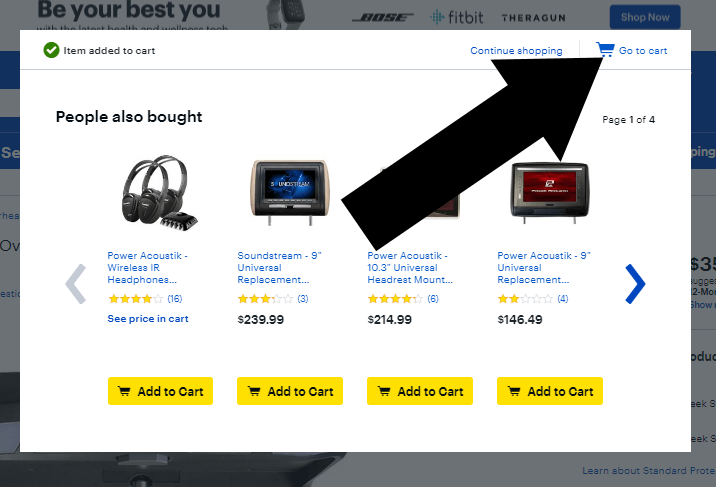The PC screenshot showcases a shopping website, though the specific company isn't identifiable. The main section of the website displays a predominantly white background with a faint horizontally-oriented greyed-out home page in the backdrop. The lone readable text in the background states, "Be Your Best You," in a flat, muted grey print. 

In the foreground, an area in the upper left corner draws attention with a white checkmark inside a green circle, accompanied by the message "Item added to cart." This section presents four distinct items, along with small thumbnails and brief descriptions. These items include:

1. **Power Acoustik Wireless IR Headphones**:
   - Price: See price in cart 
   - Rating: 4 out of 5 stars 
   - Bright yellow "Add to Cart" button

2. **SoundStream 9 Universal Replacement**:
   - Price: $239 
   - Description: Appears to be a display component, though specifics are unclear 

3. **Power Acoustik 10.3 Universal Headrest Mount**:
   - Price: $249.99 
   - Description: Detailed under an icon with a large black arrow that directs towards the upper right, indicating a "Go to Cart" section with a shopping cart icon

4. **Power Acoustik 9 Inch Universal Replacement**:
   - Price: $146.49 
   - Description: The nature of the item is ambiguous but categorized as a universal replacement part, similar to the other display component

The far right edge of the screen features a blue right arrow, likely meant for navigating to additional items on the website.